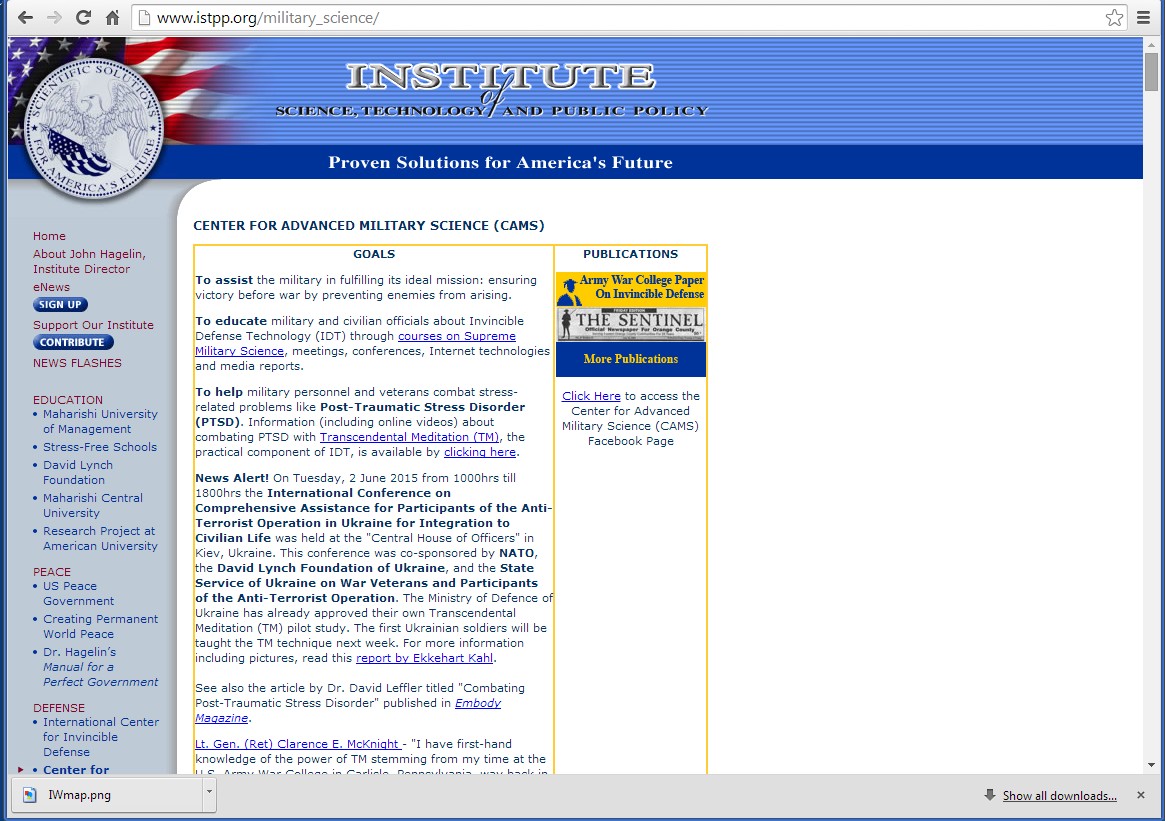The image is from the Institute of Science, Technology, and Public Policy, commonly referred to as CAMS. The primary goal of CAMS is to support the military in achieving its ideal mission by ensuring victory through the prevention of enemies before the onset of war. The image features a prominent blue box with the text "Proven Solutions for America's Future" and identifies the organization as the Center for Advanced Military Science.

The objectives of CAMS include educating both military and civilian officials about invincible defense technology through specialized courses on supreme military science. Additionally, it aims to assist military personnel and veterans in combating PTSD, offering resources such as online videos that highlight the benefits of transcendental meditation for PTSD relief.

A news alert within the image details an international conference held on Tuesday, June 2, 2015, from 10:00 AM to 6:00 PM. The event, titled "Comprehensive Assistance for Participants of the Anti-Terrorism Operation in Ukraine for Integration to Civilian Life," took place at the Central House of Officers in Ukraine. The conference was co-sponsored by NATO, the David Lynch Foundation of Ukraine, and the State Services of Ukraine for War Veterans and Participants of the Anti-Terrorist Operation.

The Ministry of Defense of Ukraine has approved a pilot study involving transcendental meditation for their soldiers, with the first group set to learn the technique the following week. The image also references an article by Dr. David Leffner on combating PTSD. 

The detailed caption provides a comprehensive overview of CAMS' mission and highlights the collaborative efforts to support veterans and military personnel internationally.